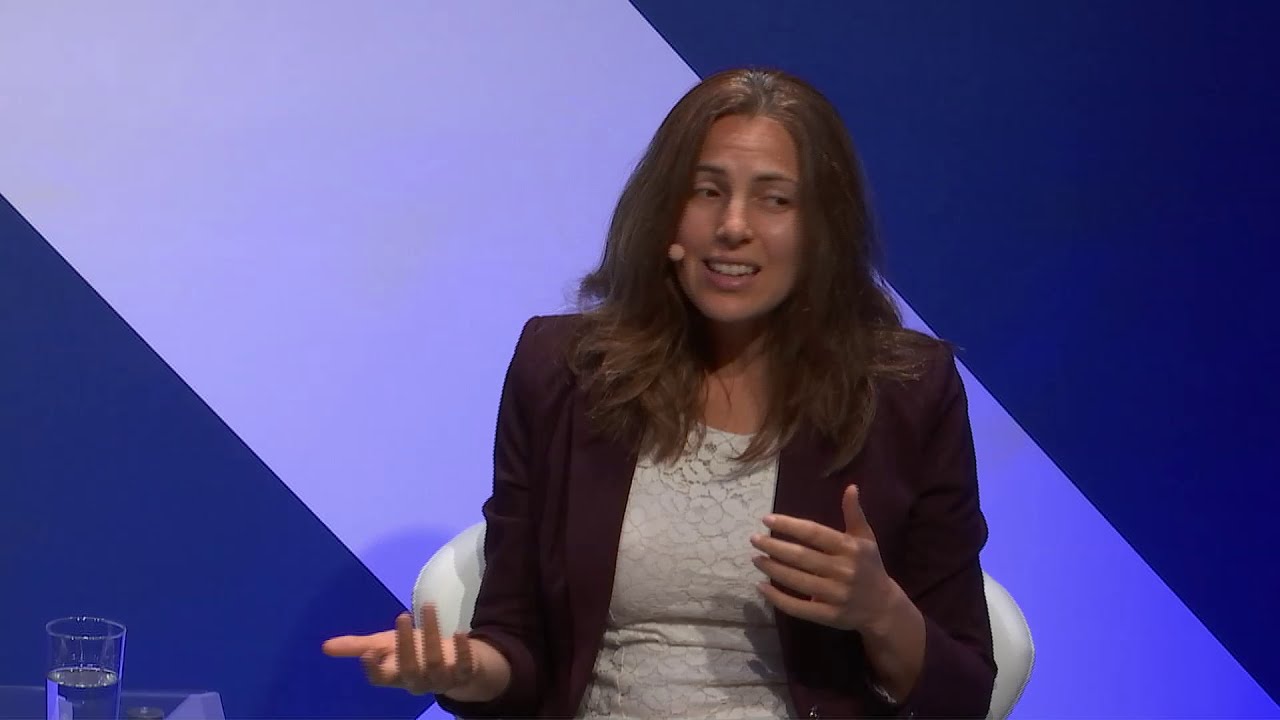This image appears to be a still from a newscast featuring a woman with long, flowing brunette hair that cascades past her shoulders. She is seated in a white padded chair and dressed in a dark suit jacket that has a brownish or purplish hue, paired with a white lacy shirt underneath. The woman is actively engaged in speaking, with her left hand raised towards her chest and her right hand palm-up near her stomach, suggesting she is in mid-sentence. Her mouth is open with teeth closed, and she is looking slightly downward to her left. A small tan microphone is visible, attached near the left side of her face. In the lower left corner of the frame, there is a small table with a glass of water. Behind her, the background features a diagonal stripe running from the top left to the bottom right in lighter blue, set against a dark blue backdrop with two darker triangular sections in the bottom left and upper right corners.